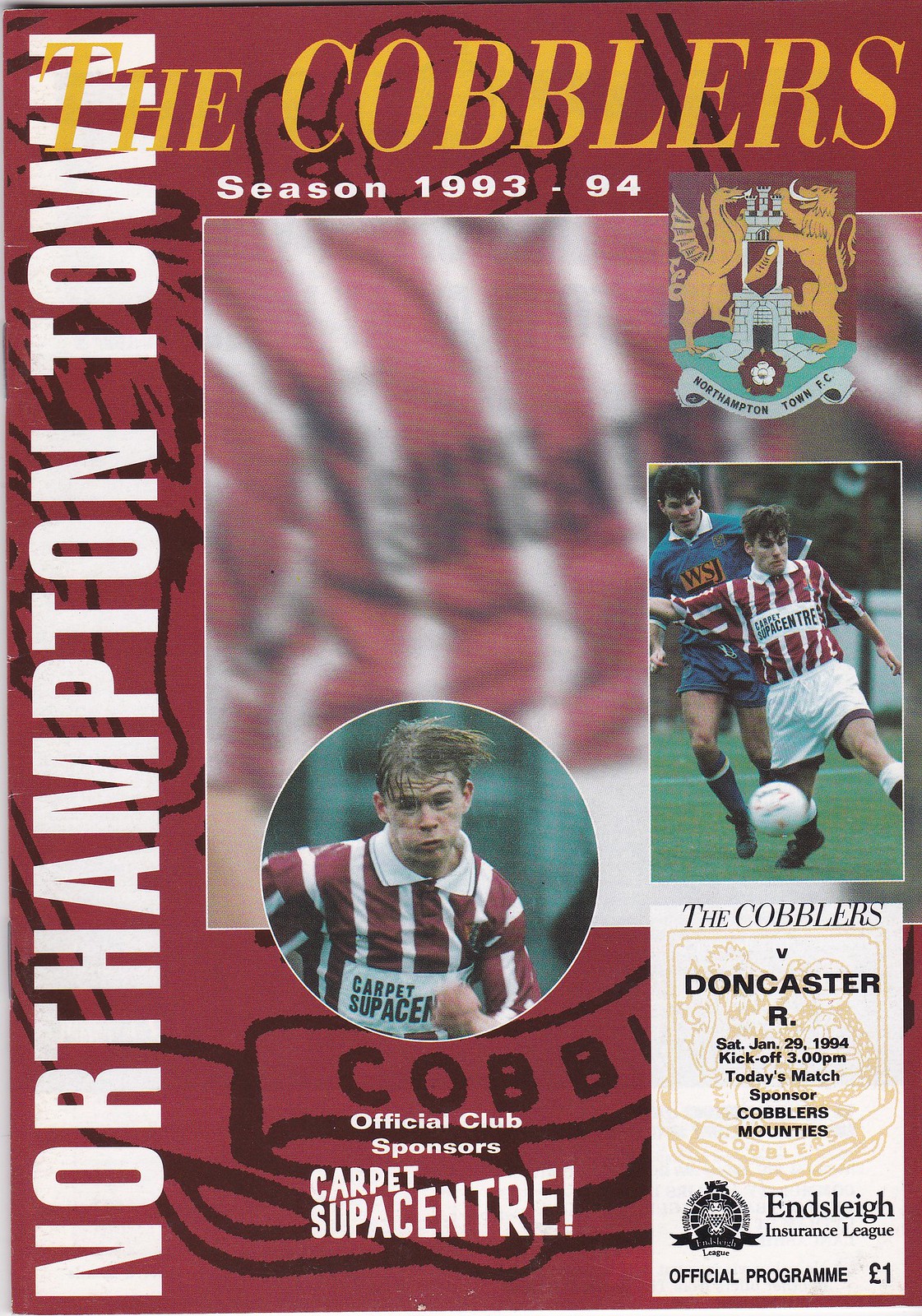The vertically aligned rectangular image is a detailed cover of a soccer magazine from the 1993-94 season. At the top in bold, all-caps yellow text, it reads "THE COBBLERS," followed by "Season 1993-94" in white print. Located centrally is a blurred square image that resembles a red and white jersey amidst a backdrop of similar hues. Dominating the center is a prominent circular close-up of a man running intensely in a red and white striped jersey with the partially visible text "Carpet Supercenter."

Additionally, a rectangular cutout overlays the background, depicting two soccer players mid-action: one in the iconic red and white jersey kicking a soccer ball, and another in a blue jersey trailing behind. At the bottom right, a rectangular section announces, "The Cobblers vs. Doncaster, Saturday, January 29th, 1994, kickoff at 3 p.m. Today's match sponsor: Cobblers Mounties."

The layout is accentuated by vertically printed, large white all-caps letters along the left side, stating "NORTHAMPTON TOWN." The cover exudes a 90s vibe with its vivid colors and dynamic design, appearing as an official program for a live soccer match, highlighted by the club's sponsor, Carpet Supercenter.